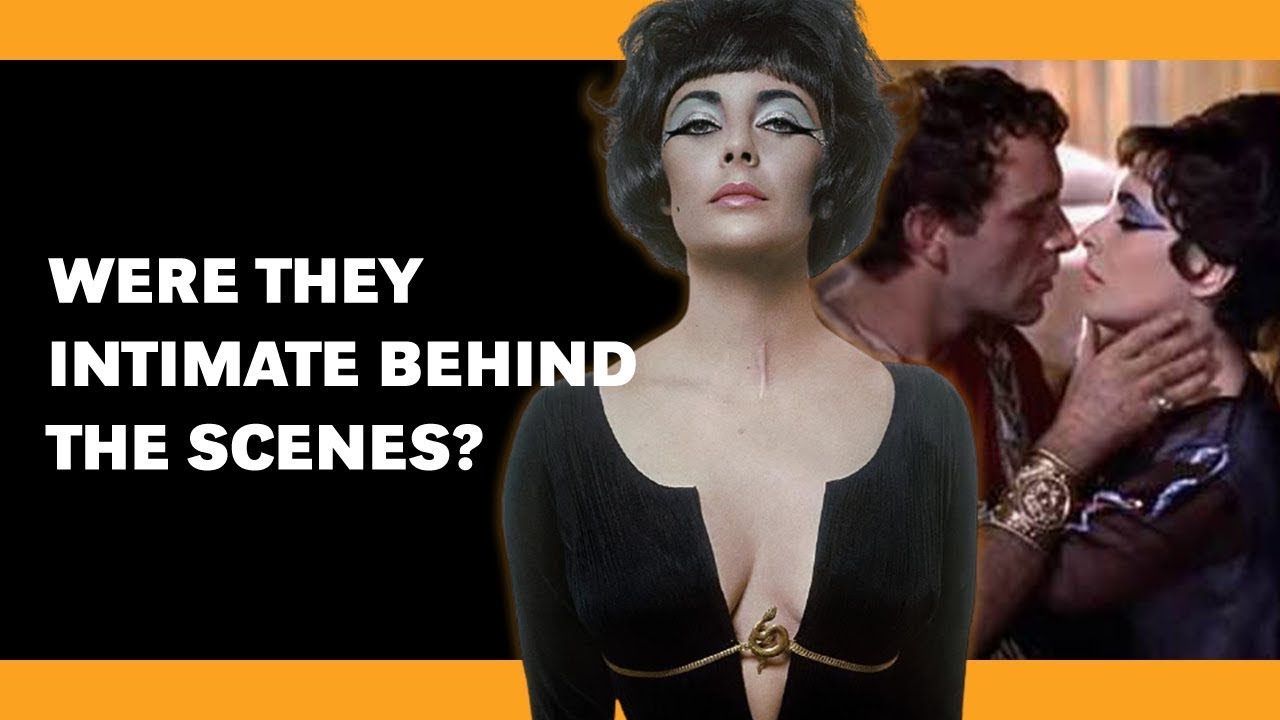The wide-framed image, likely a thumbnail for a YouTube video or website article, is bordered by bright pumpkin orange bars on the top and bottom. On the left-hand side, a plain matte black background features bold white capital letters that ask, "WERE THEY INTIMATE BEHIND THE SCENES?" The center of the image prominently displays Elizabeth Taylor adorned in her iconic Cleopatra attire, characterized by heavy blue eye shadow and dramatic black eyeliner. Her hair is styled in a bob, and she is wearing a provocatively scanty black blouse accentuated with a snake medallion just under the breasts, revealing considerable cleavage. On the right side of the image, a film screenshot shows Elizabeth Taylor, in similar attire, intimately close to Richard Burton, who is dressed as a Roman figure, perhaps Julius Caesar. They are nose to nose, with Burton's hand gently on her neck, seemingly about to kiss.